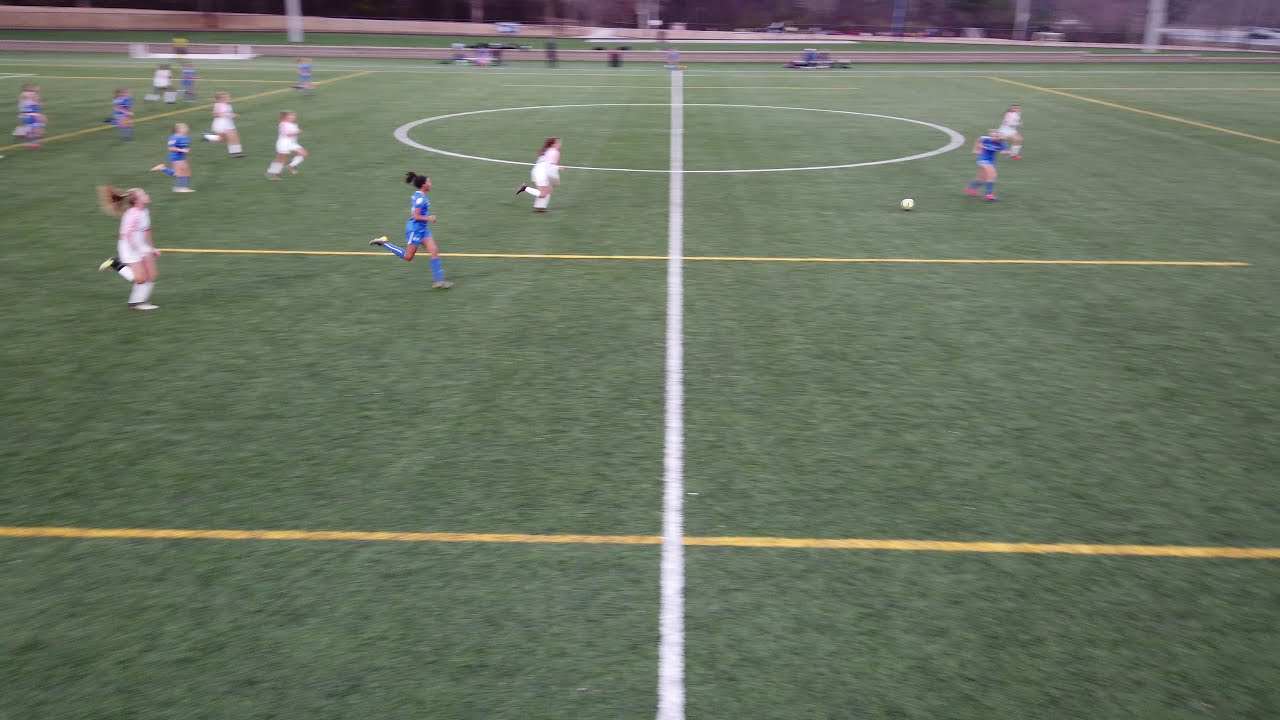This image captures a dynamic moment in a youth girls' soccer game from an aerial perspective, likely taken by a drone. The photo is slightly blurry, adding to the sense of motion as all the players are actively running across the green, grassy field. The center of the field is marked by a prominent white circle and a vertical white line stretching from top to bottom. Two horizontal yellow lines also cut across the field. Most of the players are clustered on the left side, primarily in the upper left corner, with teams easily distinguishable by their blue and white jerseys. The blue team player is seen turning towards the ball situated on the right side of the field, while other players, including two from the white team, are in pursuit. In the background, concrete structures are faintly visible, and several people can be seen on the far side of the field, possibly observing or officiating the game.